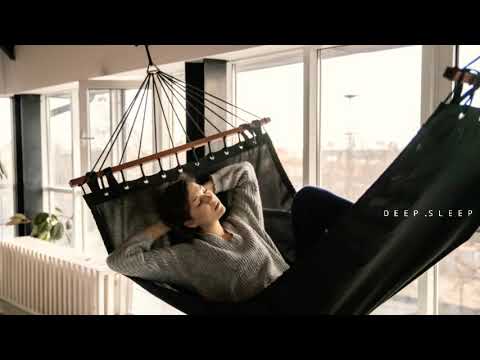The photograph captures a serene indoor setting where a woman is peacefully resting in a black, netted hammock. The hammock is suspended from the ceiling or wall, near a series of large windows that provide a glimpse of a brightly lit cityscape outside. The woman, clad in a gray sweater, has her eyes closed and her hands comfortably positioned behind her head. Her head tilts slightly to the left, and the hammock's steep angle gives an impression of precariousness, though she seems to be sleeping deeply. A sign on the right side of the image reads "DEEP. PERIOD. SLEEP." suggesting that the image might be an advertisement for the hammock. The interior of the room features contrasting wooden beams and black walls, with what appears to be a radiator or folded chairs in the lower left corner, adding depth to this cozy, urban hideaway.